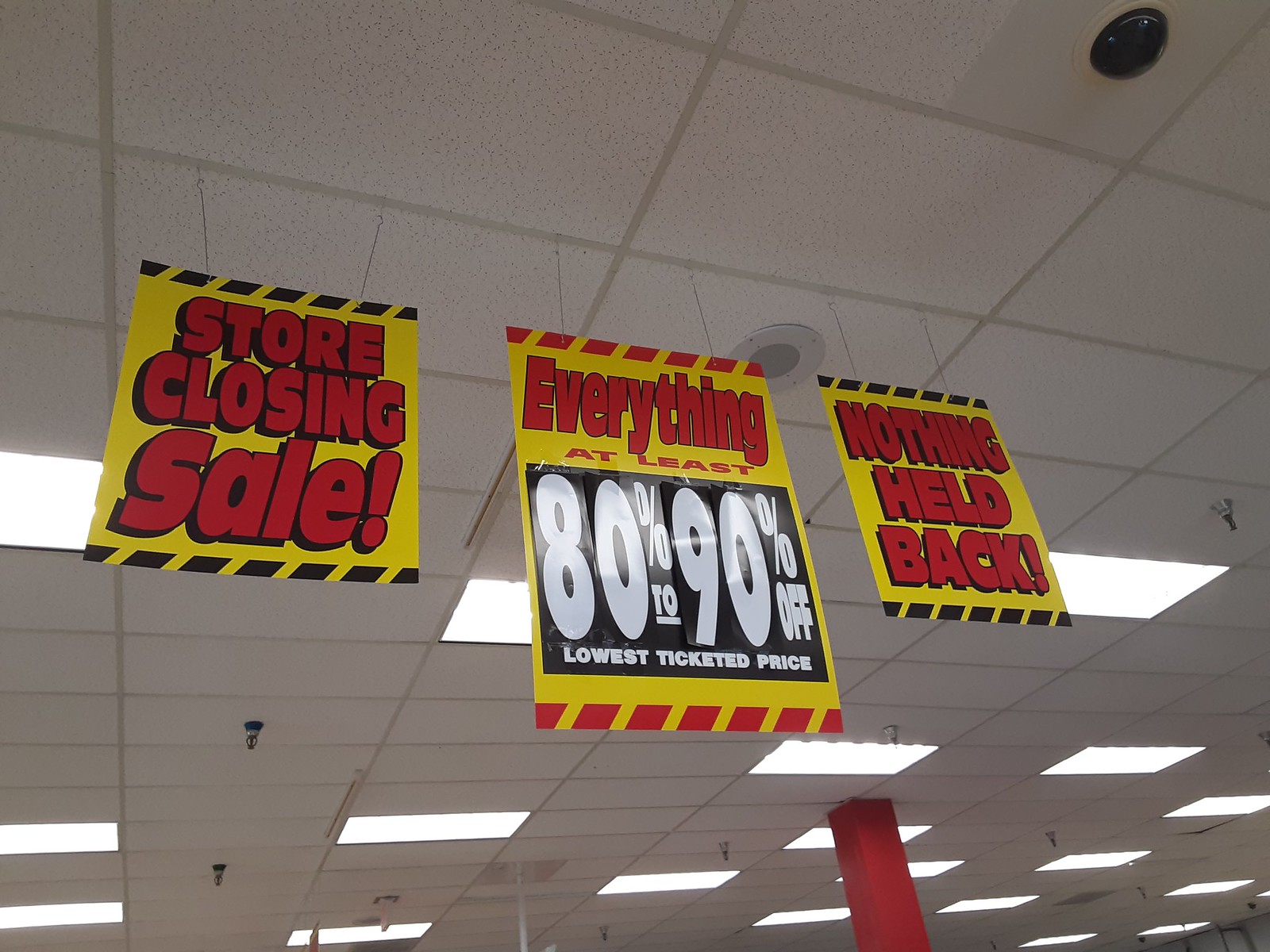The photograph captures the ceiling of what appears to be a large department store undergoing a closing sale. Dominating the view are three professionally made bright yellow signs with red block lettering. The left sign, with black trim on the top and bottom, boldly declares "Store Closing Sale!" The central sign, also the largest, features a red trim and a prominent black rectangle with white numbers, stating, "Everything at least 80-90% off lowest ticketed price." The right sign, matching the left with black trim, emphasizes "Nothing Held Back!" with an exclamation point. The drop ceiling consists of rectangular white panels interspersed with perspex light covers housing fluorescent lights, making the store brightly lit. Sprinklers for the fire system are symmetrically scattered across the ceiling, visible alongside some hanging wires and a red support pole. Additionally, a CCTV camera is noticeable in the top right corner, enhancing the store’s security.